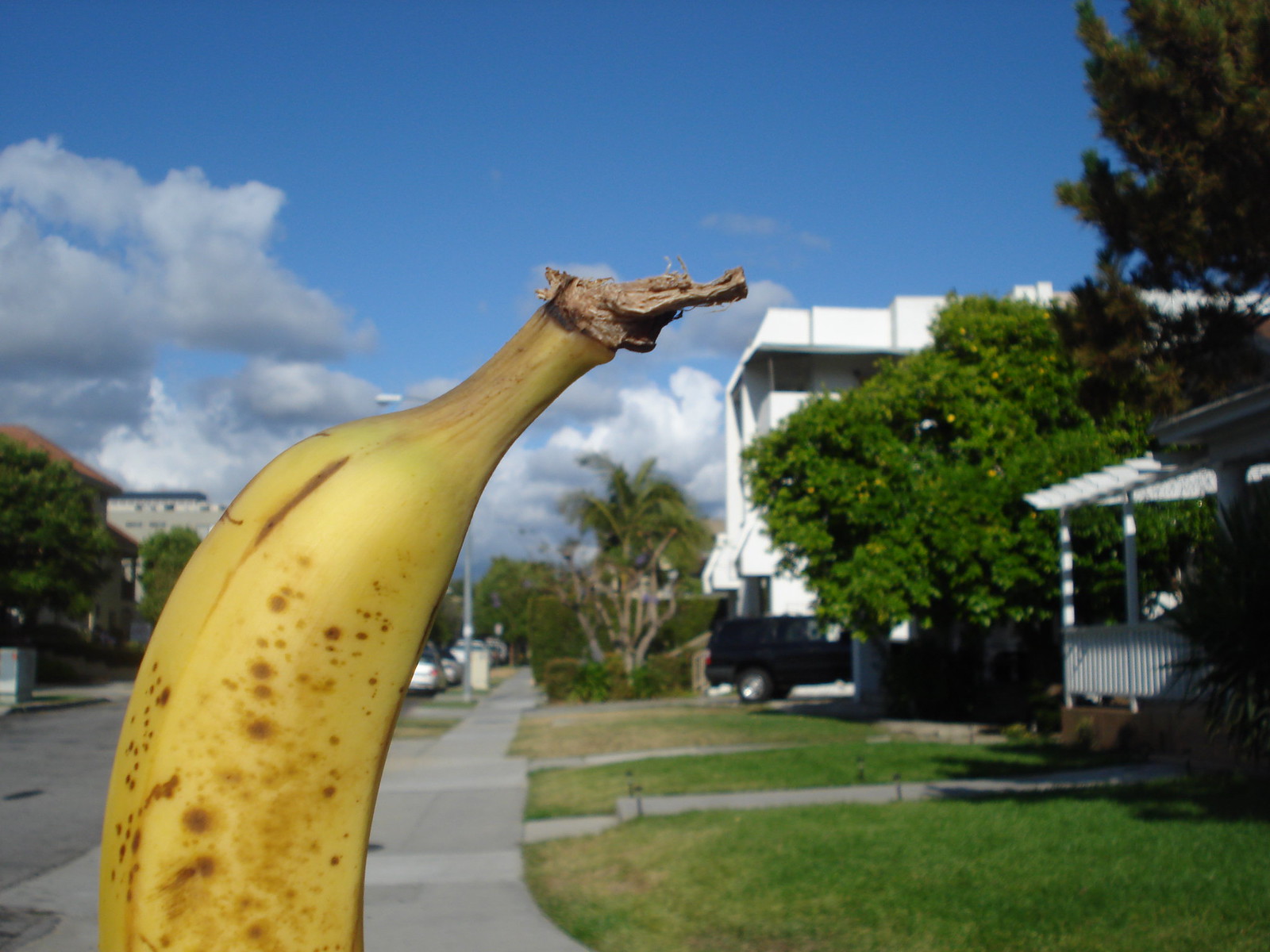The image features a prominently displayed, medium-ripe banana in sharp focus, positioned in the upper half of the frame. The banana, with a gentle upward curve and a nearly yellow hue with minimal green near the stem, displays an ideal ripening pattern with scattered brown spots. It hovers above a sidewalk in a suburban neighborhood setting. The banana's stem nearly touches the top edge of a white, two-story house, in front of which a black pickup truck or SUV is parked. Adjacent to this is another house to the right, separated by a leafy tree. In the distance, the image reveals a tall palm tree against a serene blue sky with light, wispy clouds. To the left of the banana, additional trees, a road, and a building can be seen. Three cars and a lamppost are visible in the background, portions of which peek out from behind the banana, all contributing to the illusion of depth and a whimsical overlay of natural and urban elements.